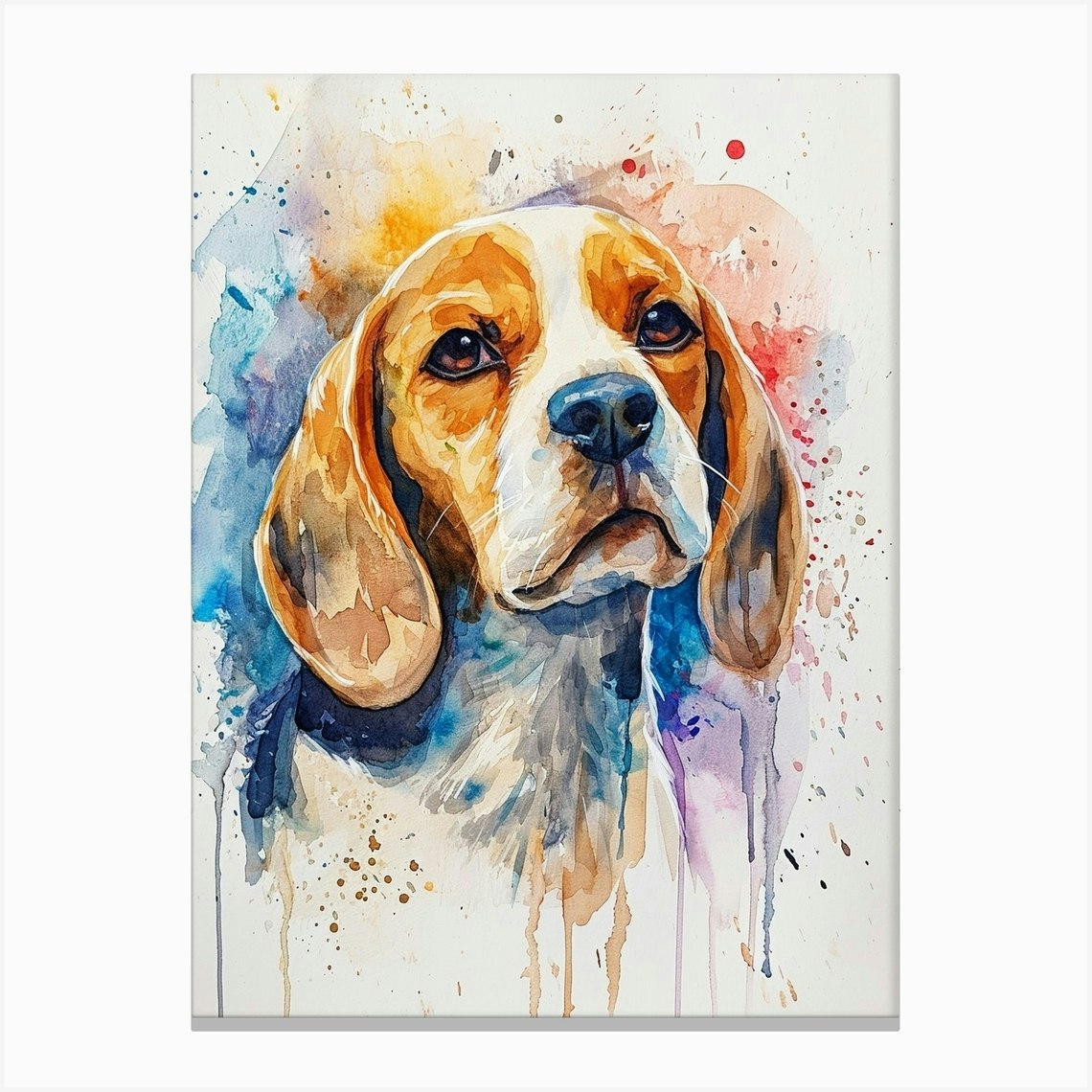This image is a digital painting designed to resemble a watercolor, prominently featuring the close-up head of a beagle or similar hound. The beagle's face, complete with a broad white stripe down to its dark nose, is marked by big brown eyes and long, droopy ears. The portrait captures the head and chest of the dog, with its head slightly tilted to the left. A mix of vibrant colors surrounds the beagle's face, creating a dynamic, drippy effect where blues, purples, reds, and yellows blend and cascade down onto the canvas. These colors give the piece a lively, splashy ambiance, suggesting the paint was purposefully splattered. The entire composition rests on a white or off-white background, enhancing the vividness of the colors. The picture mimics the appearance of being hung on a wall but is clearly a crafted digital representation.